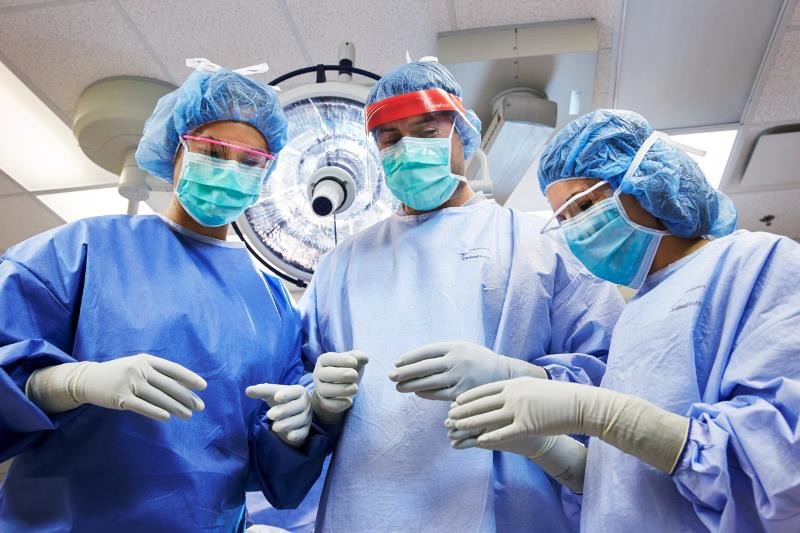This photograph captures a detailed scene inside an operating room. Three trauma surgeons are seen intently focusing on a patient who is just out of frame at the bottom of the image. Each surgeon is donned in blue scrubs and wearing light blue surgical masks that cover their faces. Their hair is neatly tucked under light blue surgical caps. The surgeon on the left, identifiable by her pink glasses, has a dark blue gown, while the center male surgeon and the third surgeon, who also wears white-rimmed glasses, are dressed in lighter blue attire. All three surgeons have white or tan-colored gloves on their hands, held up to maintain sterility as they prepare for the operation. Behind them, a large, translucent operating light hangs, illuminating the bright, white tile ceiling typical of a commercial building. There is an out-of-focus caption on the upper left corner of their gowns, likely the name of the hospital, which adds to the sense of professionalism and urgency in this vividly depicted medical setting.